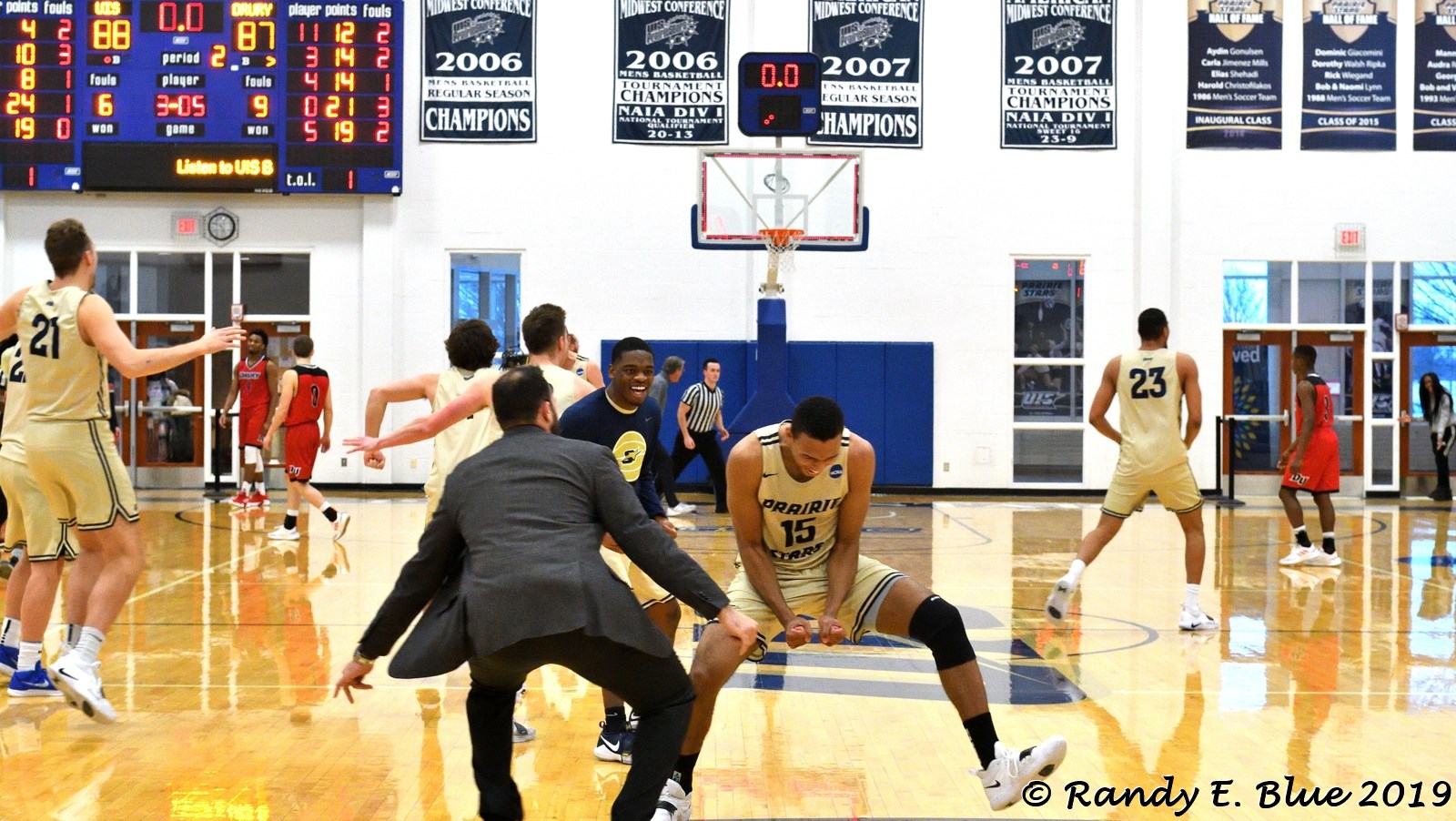This horizontally aligned rectangular image captures the exhilarating finale of a men's basketball game inside a brightly lit gym. At one end of the court, a basketball goal stands against a backdrop of blue mats propped up against a white wall, flanked by numerous rectangular banners proclaiming past championship victories from 2006 and 2007. In the upper left corner of the image, a blue digital scoreboard shows the dramatic final score of 88 to 87 with yellow and red illuminated numbers, highlighting the nail-biting conclusion of the game.

In the foreground, a poignant moment unfolds as a man in a business suit, likely the coach, bends down in front of a player wearing a white jersey with blue numbers. The player, also bent down, clenches his fists in a triumphant gesture and beams with joy, moments away from embracing the coach. Nearby, other players in white jerseys leap in celebration of their hard-fought victory. The opposing team in red jerseys with black numbers stands in stark contrast. In the lower right-hand corner, the image is captioned with "Randy E. Blue, 2019" in black text, anchoring the date and giving credit to the photographer.